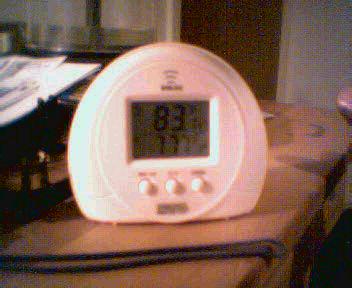In the image, we observe a severely pixelated and hazy photograph, likely taken with an old camera. The focus of the image is a white, round, and flat-bottomed smoke alarm, prominently featuring three buttons and a small screen displaying a wireless symbol. The smoke alarm is positioned on top of a wooden desk. Directly in front of the smoke alarm lies a black string or lanyard. 

The background includes a white wall and an indeterminate doorway or open entrance that appears dark and shadowy, making it difficult to discern its details. To the right of the smoke alarm on the desk, there is a black platform holding a stack of white paper. Behind this paper, a partially used set of black CD cases can be seen, with roughly one-fourth of the cases remaining in the holder.